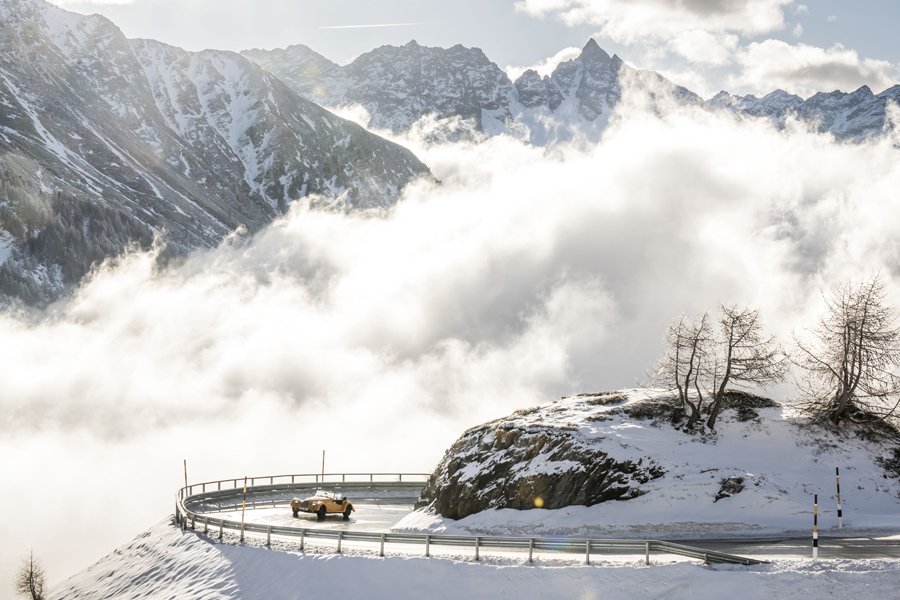The photograph captures a dramatic winter scene high in the mountains. The sky is overcast with gray and white clouds that weave through and above a majestic mountain range in the background. The mountains, appearing dark gray and grand, are partially obscured by a thick blanket of fog and clouds, hinting at a high elevation. In the mid-ground to the left, another layer of mountains adds depth to the landscape.

Dominating the foreground, a curved paved road forms a U-shape around a prominent, round rock outcropping that is covered in snow. This outcropping is sparsely dotted with barren trees that have shed their leaves, typical of the harsh winter season. The road features a guardrail, necessary for the steep and treacherous mountain terrain, and a fence along the cliff side. A classic retro-style yellow convertible, reminiscent of mid-20th century sports cars, navigates the winding road, adding a touch of color and life to the monochromatic scenery. The image beautifully conveys the solitude and grandeur of a high-altitude winter landscape.